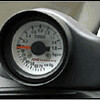A tightly cropped, low-resolution image focuses on a small speedometer, measuring approximately 100 pixels by 100 pixels or smaller. The speedometer appears to be part of either a bike, a sports car, or possibly a foreign car, featuring a distinctive design not typically embedded into a dashboard. The surrounding area showcases gray plastic with a texture mimicking a faux leather grain. The speedometer's dial has a white face with black numbers and markings, although the poor quality of the image makes the numbers indistinguishable. A red needle sits in the center, poised to indicate the speed. The photo is quite dark, with minimal light filtering in from a windshield in the background, failing to illuminate the scene adequately. The speedometer is encased in a round, bubble-like console, making it stand out within the confined frame.